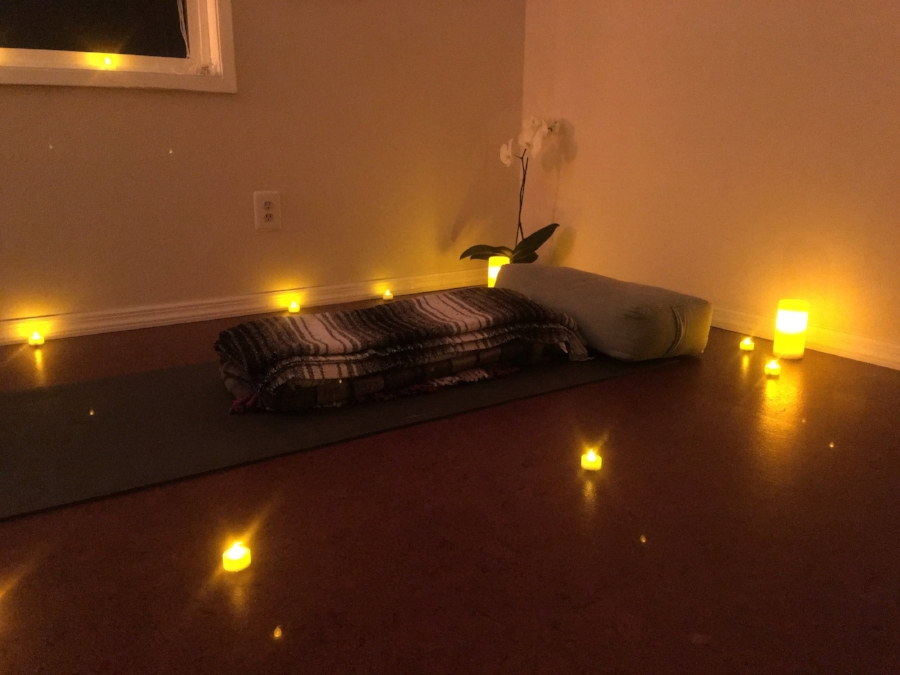The image depicts a small, dimly lit room with a dark wooden floor and white walls. In the corner of the room, under a window with an electrical outlet below it, lies a green yoga mat adorned with a neatly folded brown and white striped wooly blanket and a pillow. Surrounding the yoga mat are about ten yellow lit candles, creating a serene and romantic ambiance. Beside the mat, in the furthest corner of the room, there is a vase holding a single white flower with stemmed flowers. Additionally, two lamps are positioned on each side of the pillow, further enhancing the tranquil setting. The overall arrangement suggests a simple but inviting space designed for relaxation or meditation.